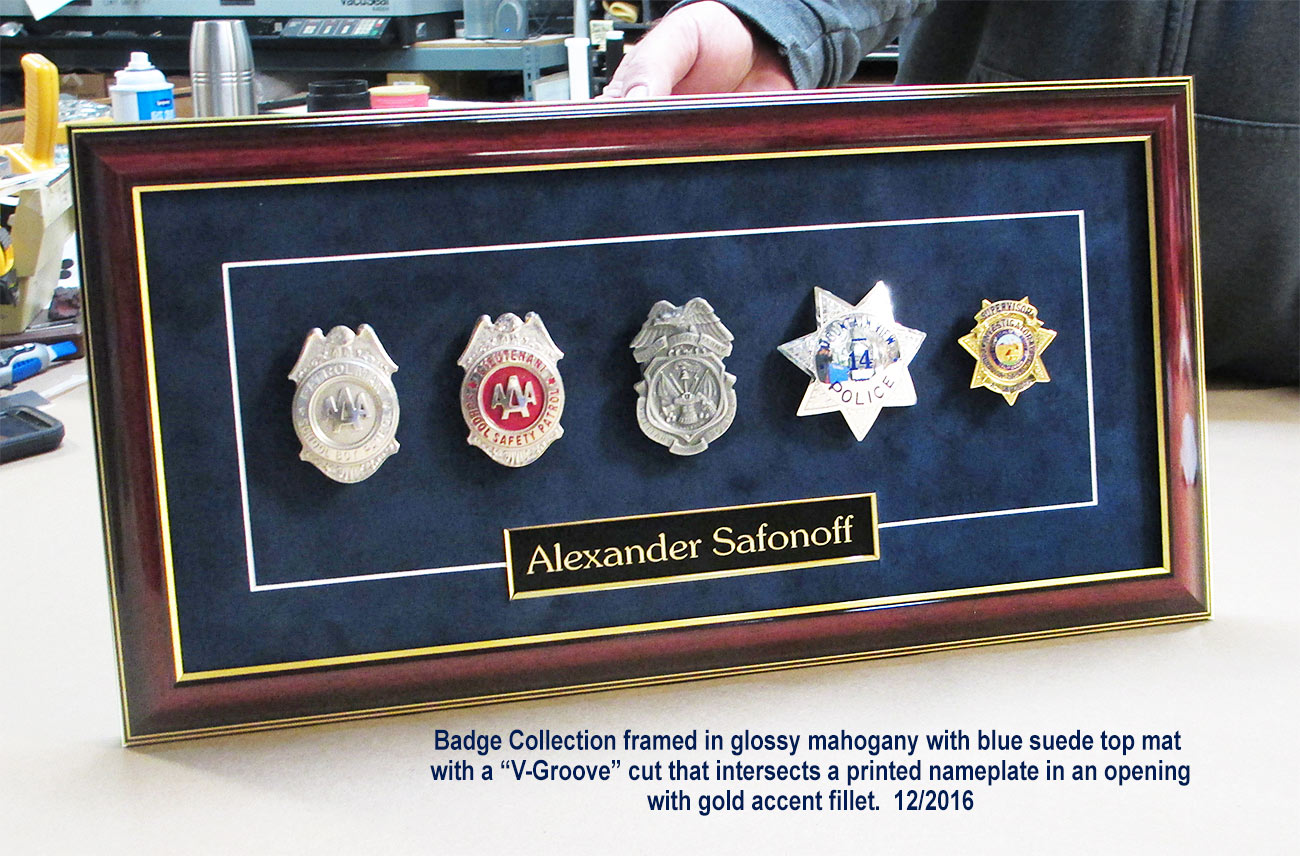The image is a detailed color photograph of a meticulously crafted framed display, commemorating a collection of police badges. The frame, made with glossy mahogany, houses five distinct badges against a backdrop of blue suede. The collection, which includes three shield-shaped badges with wing designs at the top, and two star-shaped badges – one silver, one smaller and gold – is complemented by a v-groove cut mat. At the center, beneath the badges, is a prominent printed nameplate with the gold-accented name "Alexander Safonov." At the lower right corner of the display is a descriptive text: "badge collection framed in glossy mahogany with blue suede top mat with V-groove cut that intersects a printed nameplate in an opening with gold accent fillet. 12-2016." The frame rests on a light-colored table, possibly near various tools and personal items indicated in the background, such as a thermos and cleaning supplies, lending an environment of everyday utility to this elegant display.